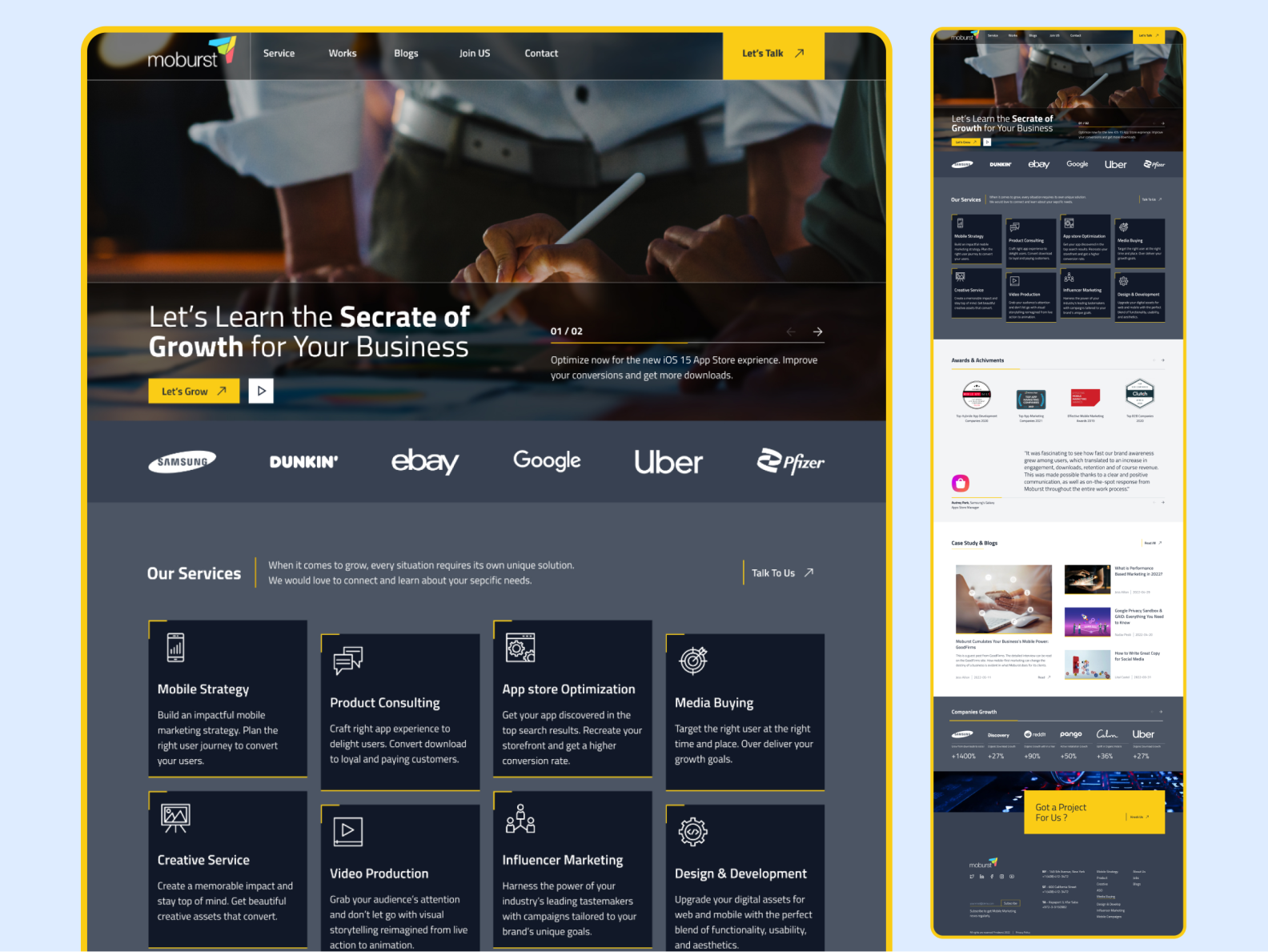The image titled "Mo Burst" is a detailed representation of a digital platform interface, featuring two distinct layouts side by side. On the left, there appears to be a website or an iPad version of the interface, while the right side showcases what looks like the complete homepage of the website, inclusive of the landing page as well as the sections visible upon scrolling down.

Both interfaces are framed with a yellow border and prominently display the "Mo Burst" logo in the upper left corner. The top navigation menu includes options such as Service, Works, Blogs, Join Us, and Contact, along with a yellow "Let's Talk" button. The left side of the layout includes an image of a person with a white pen, appearing to write something, with another individual in a suit in the background. Accompanying text reads, "Let's learn the secret of growth for your business" and another yellow button labeled "Let's Grow".

On the right side of the interface, there's a section promoting optimization for the new iOS 15 App Store, urging users to "Improve your conversations and get more downloads." Below this, logos of prominent companies such as Samsung, Dunkin, eBay, Google, Uber, and Pfizer are displayed, followed by a series of boxes detailing various services the company offers.

The right layout further extends to a white area populated with additional icons, and at the bottom, a darker section with a call-to-action button that says "Got a project for us?". The detailed design and structured elements provide a comprehensive overview of the services and capabilities offered by Mo Burst, ensuring an engaging user experience.